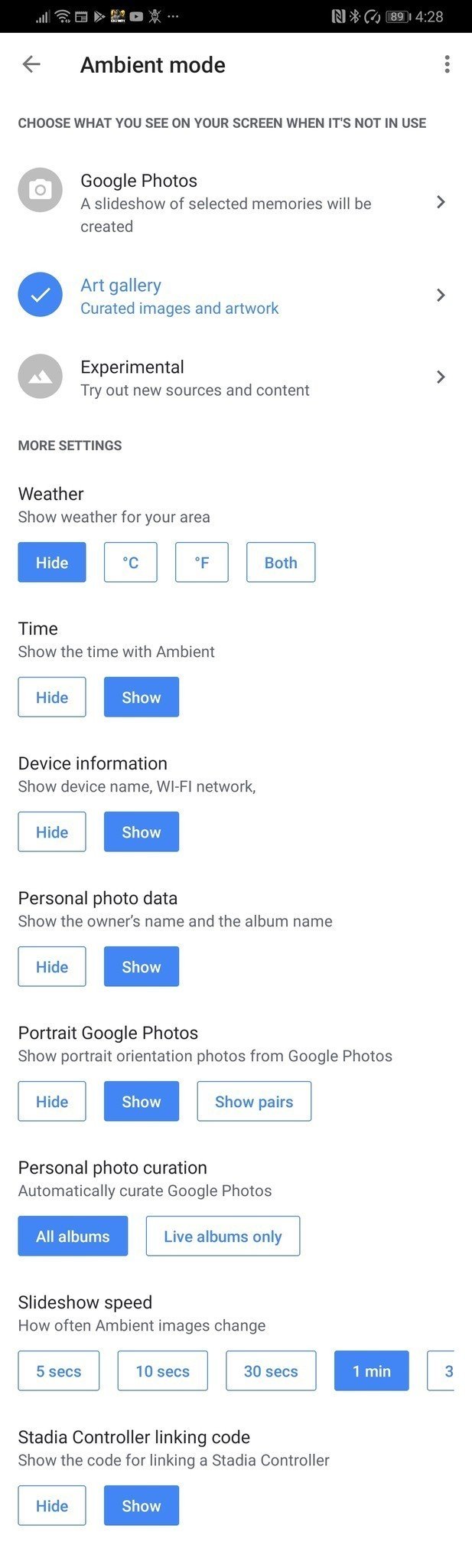The image is a vertically rectangular screenshot from a mobile phone, exhibiting some distortion in the text. At the top, there's a narrow black banner displaying phone icons for Signal strength, Battery level, and Wi-Fi connection. The time appears to be 4:28. Below this banner, the background is predominantly white, with a heading titled "Ambient Mode," accompanied by the subtitle, "Choose what you see on your screen when it's not in use."

Following the heading is a vertical list with selectable items:

1. **Google Photos**
2. **Art Gallery** (currently selected)
3. **Experimental** - with a description, "try out new sources and content."

Further down, there are additional settings options:
- **Weather** - button for "Hide"
- **Time** - button for "Hide"
- **Device Information** - button for "Hide"
- **Personal Photo Data** - button for "Hide"
- **Portrait Google Photos** - button for "Hide"
- **Personal Photo Curation** - options for "All Albums" or "Live Albums Only"
- **Slide Show Speed** - button for "Show"
- **Stadia Controller Linking Code** - button for "Show"

Each of these settings offers a "Hide" or "Show" button except for Personal Photo Curation, which provides choices between "All Albums" and "Live Albums Only".